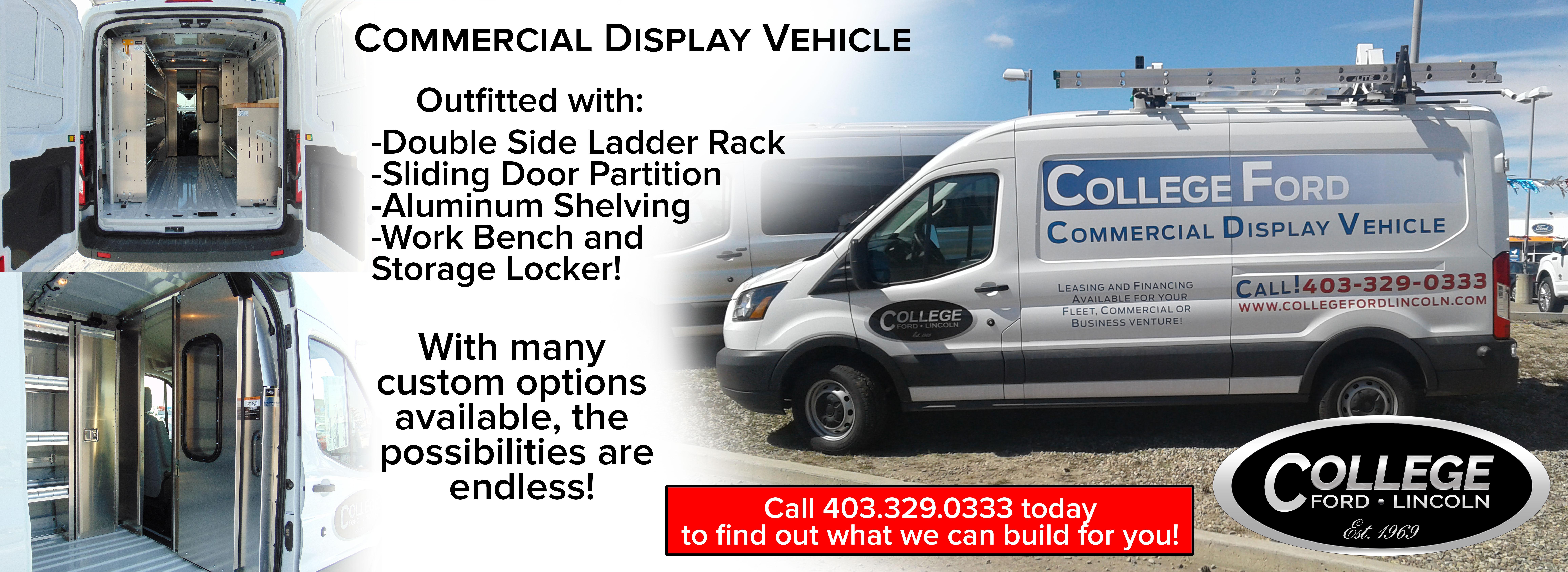The advertisement showcases a College Ford Lincoln commercial display vehicle, established in 1969. On the left side, there are two images of the van's interior from different perspectives, highlighting features like a double side ladder rack, sliding door partition, aluminum shelving, workbench, and storage locker. The text emphasizes that many custom options are available, making the possibilities endless. The right half prominently features a side profile of the van bearing the label "College Ford Commercial Display Vehicle." Smaller text beneath this label mentions leasing and financing availability for fleet, commercial, or business ventures, urging viewers to call 403-329-0333 or visit www.collegefordlincoln.com. A red banner underneath the van reiterates the contact number and encourages customers to inquire about custom builds.